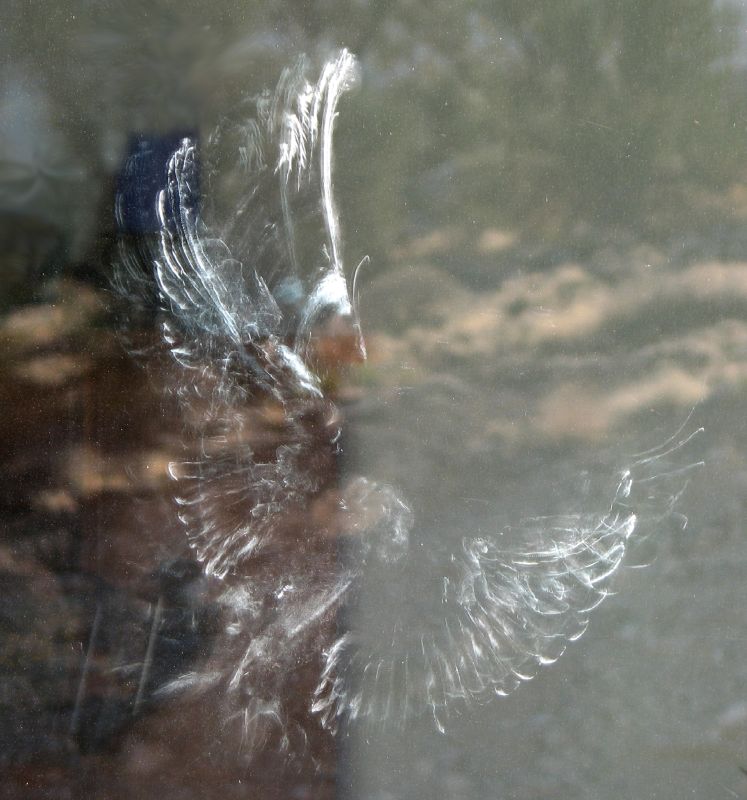The image depicts a bird resembling a quail, identified by a high feather extending above its forehead, in mid-flight with its wings expanded. The bird's wings exhibit a striking black and white pattern while its head is a vibrant orange, adorned with a white ring around its neck. The bird appears to be hovering over water, evidenced by its reflection below. The background features a blurred green foliage, suggesting an outdoor setting. Despite some blur and the possibility of the image being taken through a dingy glass surface or being a drawing, the scene captures the dynamic motion of the bird with a sense of movement that hints at multiple or reflected images of its flapping wings.